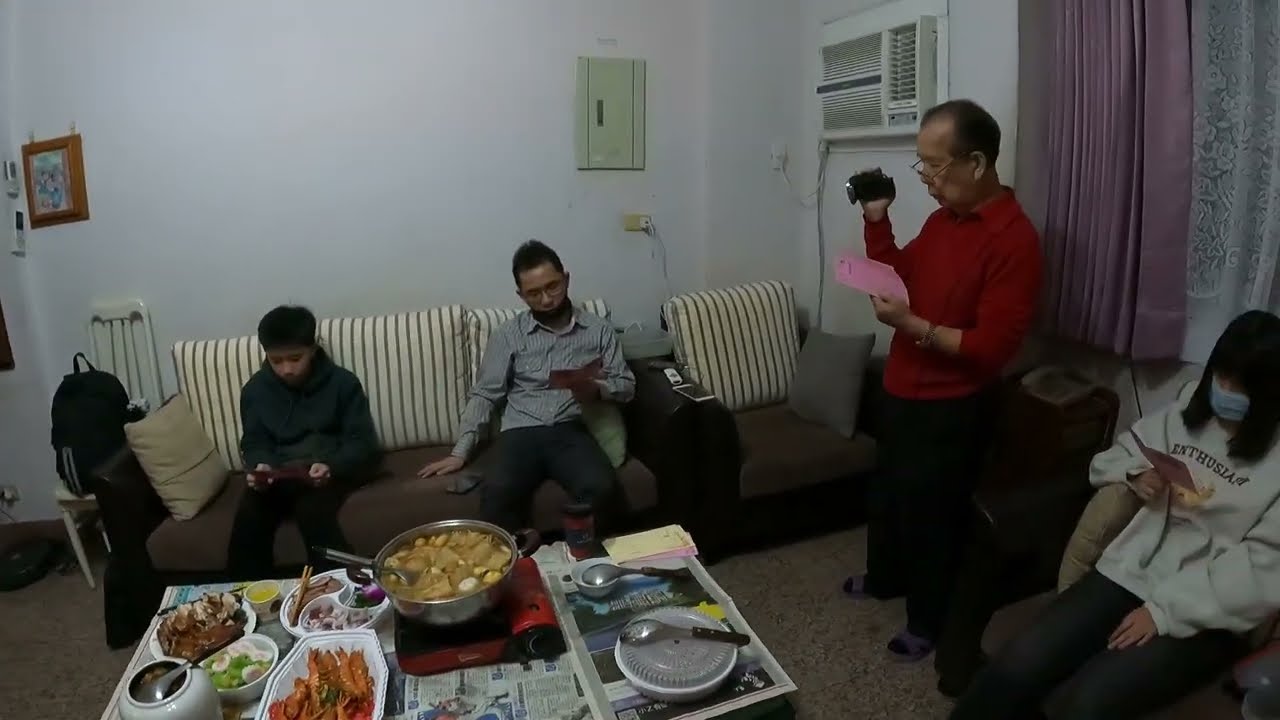In the cozy living room with white walls, an air conditioner mounted on the right, and purple drapes, a family of four of Asian descent is gathered around a table laden with a variety of Asian-style dishes, all set atop newspapers to catch any spills. Two men are seated on a couch on the left; the younger one is engrossed in what looks like a video game, while the older man beside him reads from a piece of paper. To their right stands another man in the center of the picture, holding a camcorder in his right hand and studying a pink manual with his left. Lastly, a woman sits to the far right, also reading from a pamphlet. The scene captures the warmth and togetherness of the family as they all appear focused on their respective papers, possibly instructions for a shared task or event.